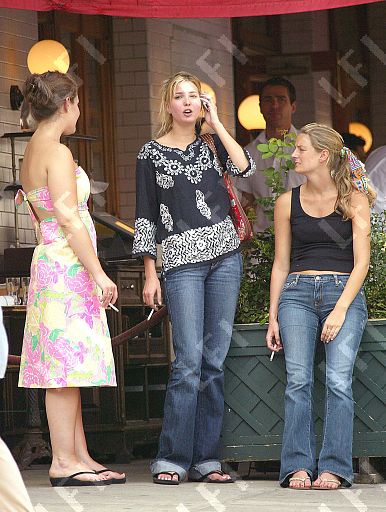In this detailed picture, three women are standing outside near a green planter and green bushes, with glowing yellow round lights in the background. To the left, a lady in a strapless white dress with pink and green flowers, black flip-flops, and her hair pulled up in a bun, stands facing to the right while looking toward a man with black hair and a white shirt in the background. She is smoking a cigarette, held down by her side in her right hand. 

The woman in the middle is dressed in a 70s-style blue shirt with flared sleeves and flowers, paired with blue jeans that look like bell-bottoms. She has long hair with brown and blonde streaks, wears white flip-flops, and has a paisley ribbon tying back her hair in a ponytail. She is also holding a cigarette and appears to be engaged in a phone call with a red purse slung over her shoulder.

To the right, the third woman is sitting on a planter box holder, showcasing a black tank top that slightly exposes her midriff, and blue jeans. She sports black sandals, holds a cigarette, and like the others, has long blonde hair tied back into a ponytail. The ensemble is framed by a setting that resembles a restaurant or stage, emphasizing their relaxed, candid posture in a social scene.